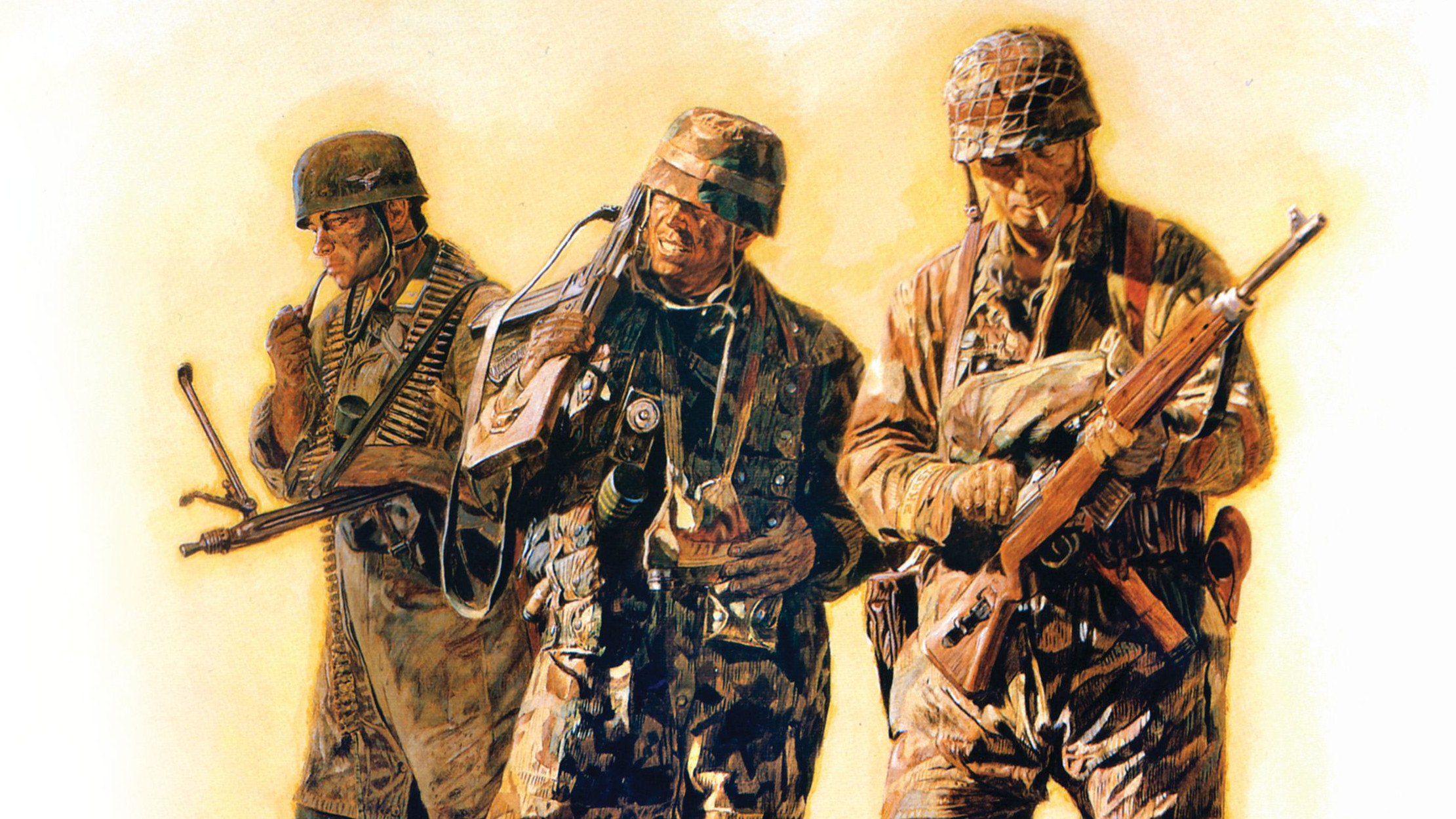In this illustration of a painting, three soldiers stand in the foreground against a hazy, swirled mustard-yellow and white background, evoking a sense of rugged militarism. Each soldier is clad in a strange camouflage pattern that combines brown, green, and grayish tones, somewhat unconventional and almost blending into the yellowish backdrop. Their faces are worn and dirty, evidencing time spent in harsh conditions.

The soldier on the left, slightly set back, puffs on a pipe while facing the left. He has a rifle slung over his left shoulder and an ammo belt draped around his neck. This soldier is looking off into the distance with a contemplative expression. 

The central figure, positioned between the other two, carries his rifle over his left shoulder and grasps onto his ammo straps. He holds a camera hanging from his chest and appears to be squinting or grimacing due to the light, exuding a stressed demeanor. 

The rightmost soldier, who is closest to the viewer, is depicted in the act of loading his rifle. He has a cigarette fixed in his mouth and looks down intently at his gun, focusing on the task at hand.

The overall scene captures the diverse and focused stances of the soldiers, brought together in a vivid, yellow-toned tableau that highlights both the surreal and gritty aspects of military life.